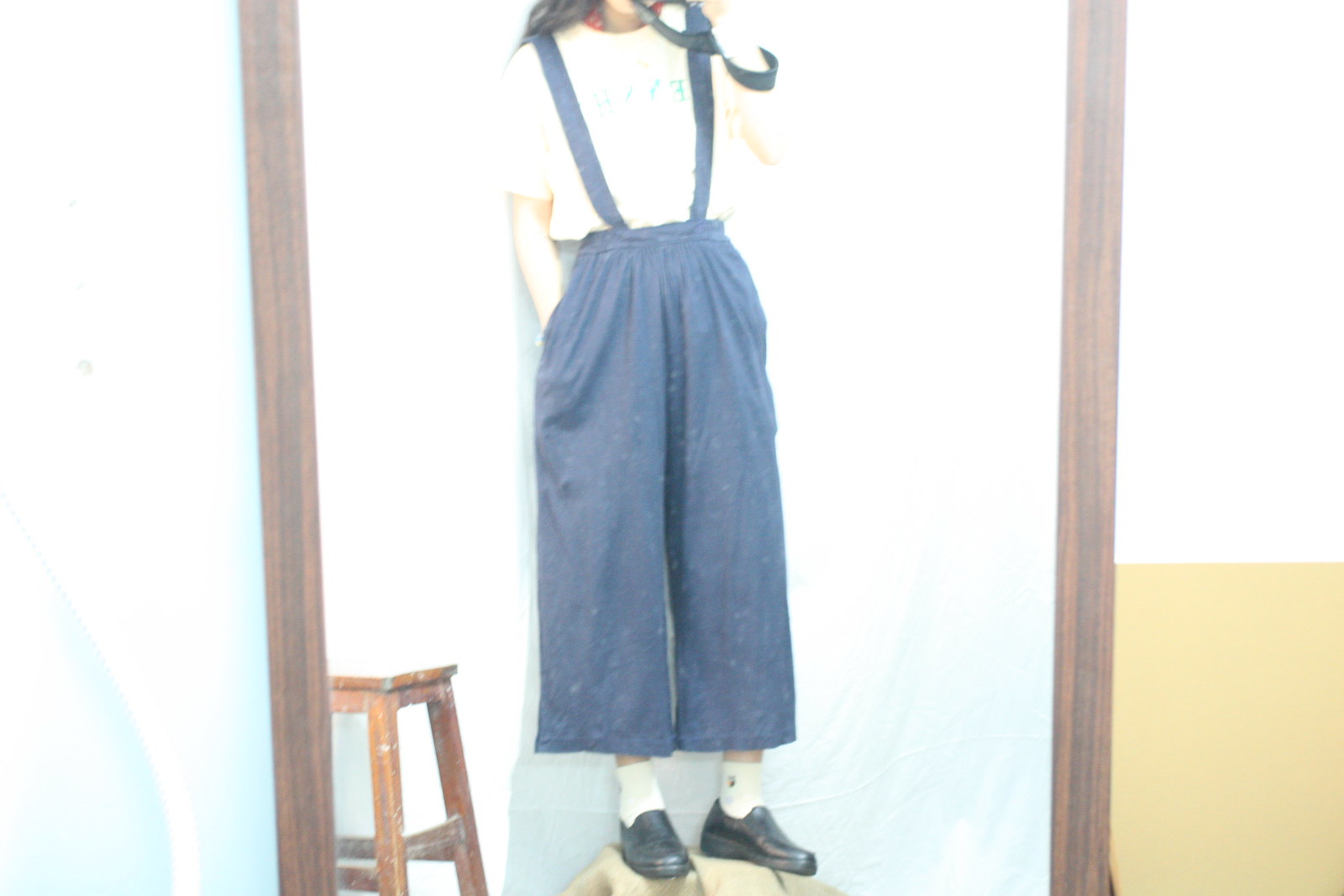The photograph captures the reflection of a girl taking a selfie in a mirror with a dark brown wooden frame. The mirror is centrally positioned with white walls surrounding it. In the reflection, the girl's image is cut off at the neck, revealing her long hair flowing to the side. She is dressed in blue dungarees with wide-legged trousers, held up by suspenders, and a white short-sleeved t-shirt with faint, unclear light blue text. She has one hand in the deep pocket of the dungarees while her other hand, likely holding a camera strap, is raised. She wears short white socks and black closed-toe shoes, standing on a light brown stool which appears to have a fabric covering. The bottom of her trousers nearly reaches her ankles, leaving a small portion of her legs visible. The image is well-lit and detailed, offering a casual yet insightful glimpse into her attire and the surrounding space.